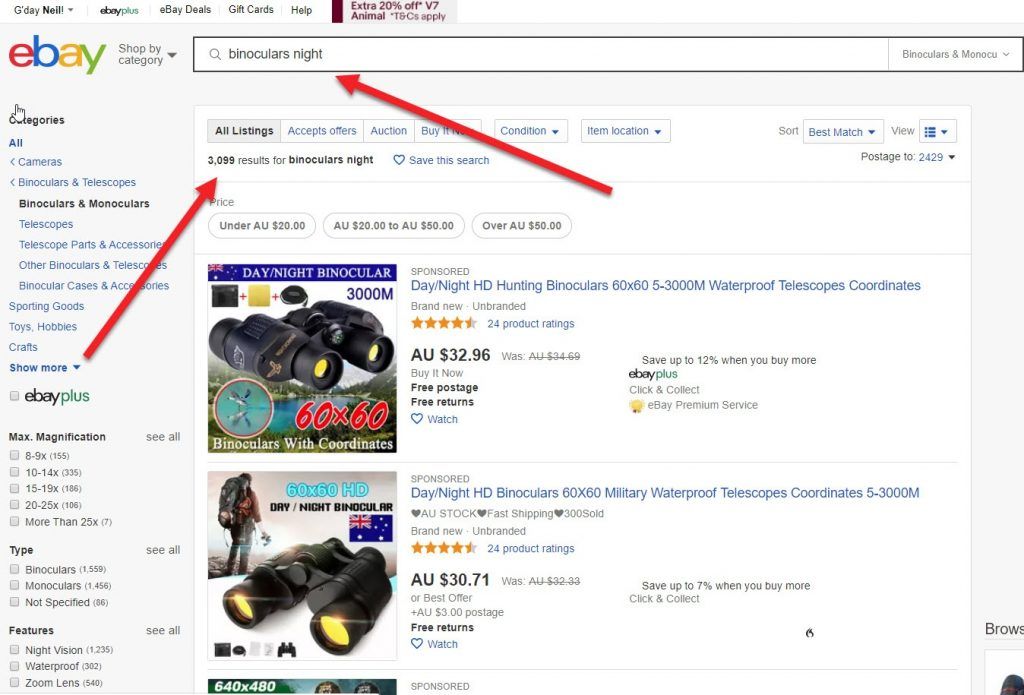A screenshot depicts a user searching for "binoculars night" on eBay's desktop version. The search results show two sponsored products at the top. The first product is titled "Day/Night HD Hunting Binoculars 60x65 - 3000m Waterproof Telescopes," priced at AUD 32.96. The image accompanying this listing showcases the binoculars in an outdoor setting near a serene lake. The second product, slightly cheaper by a few Australian dollars, is labeled "Military Binoculars" and features an image of a person looking into the distance from a snowy ski slope.

In addition to the product listings, the screenshot includes part of a third sponsored product barely visible at the edge of the view. The typical eBay site layout is present, complete with a search bar at the top where the user entered their query, and various filtering options and subcategories listed on the left side. Additionally, there are arrows on the screenshot pointing to the search bar and the number of results generated.